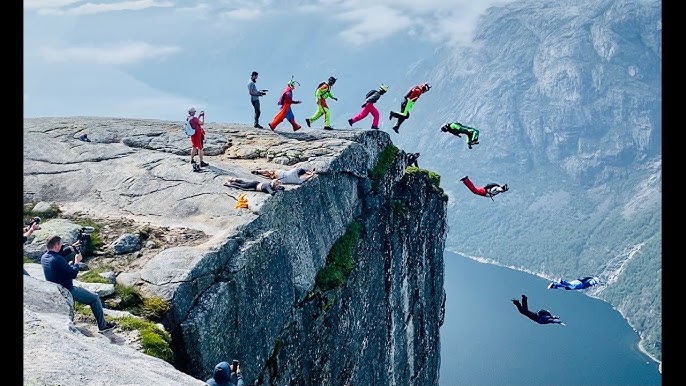In this vivid and dynamic color photograph, a group of about nine to ten people are captured in the exhilarating act of skydiving off a sheer rock cliff. The image, set in landscape orientation, vividly portrays the action against a dramatic natural backdrop. The participants are adorned in bright neon-colored protective suits, with parachutes strapped to their backs, forming a striking contrast against the rugged rock face centered in the frame. Several individuals are already airborne, showcasing their descent towards the river far below, while others are poised mid-jump or still running towards the edge in a single-file line.

The scene includes three distinct photographers: one in the rear on the left side, another reclining against a rock at the bottom left, and a third individual closer to the jumpers, capturing every moment of this daring plunge. The far distance of the image reveals additional mountain ranges descending into a floral or grassy area that meets the riverbank. The composition suggests a blend of representational realism and drone photography, capturing the essence of the adventurous leap framed by the vast and awe-inspiring landscape. The photo exudes a sense of thrill and highlights the meticulous order of the jumpers, enhancing the overall dynamism of the scene.